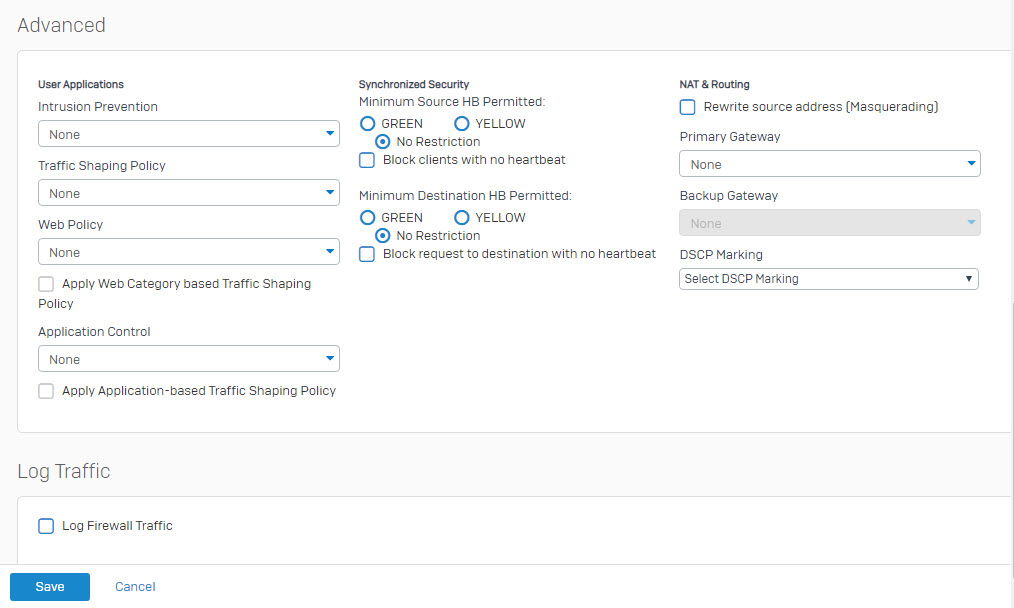This partial screenshot showcases the admin section of an IT application, framed against a grey background. Dominating the top left is the word "Advanced" in large grey letters, setting the stage for various settings and configurations.

Beneath this, a significant white box is segmented into distinct sections:
- The first section is titled "User Applications" in bold black letters. This segment includes multiple configuration options:
  - "Intrusion Prevention," accompanied by a drop-down box set to "None."
  - Below, "Traffic Shaping Policy" also features a drop-down box currently set to "None."
  - "Web Policy" follows the same pattern, set to "None."
  - Adjacent to an unclicked checkbox is the directive, "Apply web category-based traffic shaping policy."
  - Lastly within this section, "Application Control" is visibly set to "None," with an additional unchecked box reading, "Apply application-based traffic shaping policy."

At the center top, "Synchronized Security" is prominently labeled in bold black letters, detailing:
  - "Minimum Source HB Permitted" follows, listed alongside three clickable bubbles in green, yellow, and labeled "No Restriction," with the latter being selected.
  - A checkbox stating "Block clients with no heartbeat" is not selected.
  - Further below, "Minimum Destination HB Permitted" is detailed with three clickable options, again with "No Restriction" selected.
  - Another checkbox specifies "Block requests to destinations with no heartbeat," which remains unchecked.

To the right, "NAT and Routing" is marked in bold black letters. This section comprises several settings:
  - A checkbox for "Rewrite source addresses" (noted as "Masquerading") is not checked.
  - Options for "Primary Gateway" and "Backup Gateway" both display "None," with the latter box being greyed out.
  - "DSCP Marking" selection is noted, currently set to "Select DSCP Marking."

In the lower left, under a header reading "Log Traffic," the upper portion of another white box is visible though cut off from the screenshot.

This screenshot captures a variety of administrative controls and their current configurations within the application, illustrating both available and disabled options in a detailed manner.